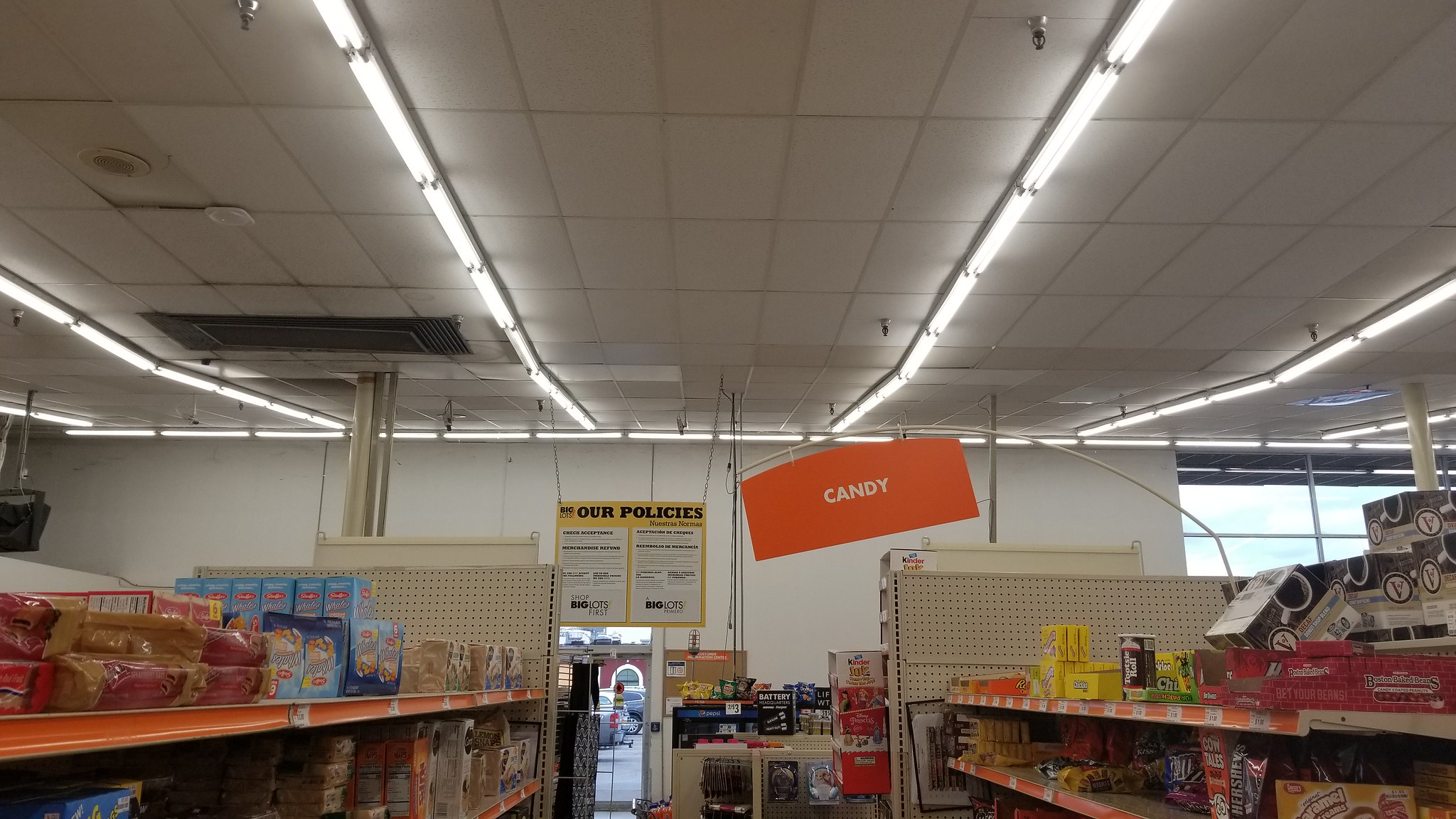The image depicts the interior of a market, likely a mom-and-pop store rather than a large supermarket, given its somewhat disheveled appearance and limited product variety. The ceiling is lined with acoustical tiles and rows of fluorescent lights that traverse the entire store. The walls are white and feature several beige shelving units with orange trim. Products are often displayed with small price stickers, although the exact pricing is unreadable. On the left side, there are shelves stocked with bread in plastic bags, various boxed products, and possibly items like flour. The right side showcases an orange box, yellow boxes, coffee pod boxes, and a container likely filled with Tootsie Rolls. Toward the back, the shelves continue, displaying candies and more boxed goods. Above the aisles, hanging signs draw the eye: a bright orange sign with "candy" written in red, and another on a yellow background that says "our policy" near a glass door leading outside, revealing a view of the parking lot. The store's shelving ends in pegboards, enhancing the utilitarian atmosphere. Despite the "candy" sign, the aisle it marks seems to contain various food items rather than just candy.